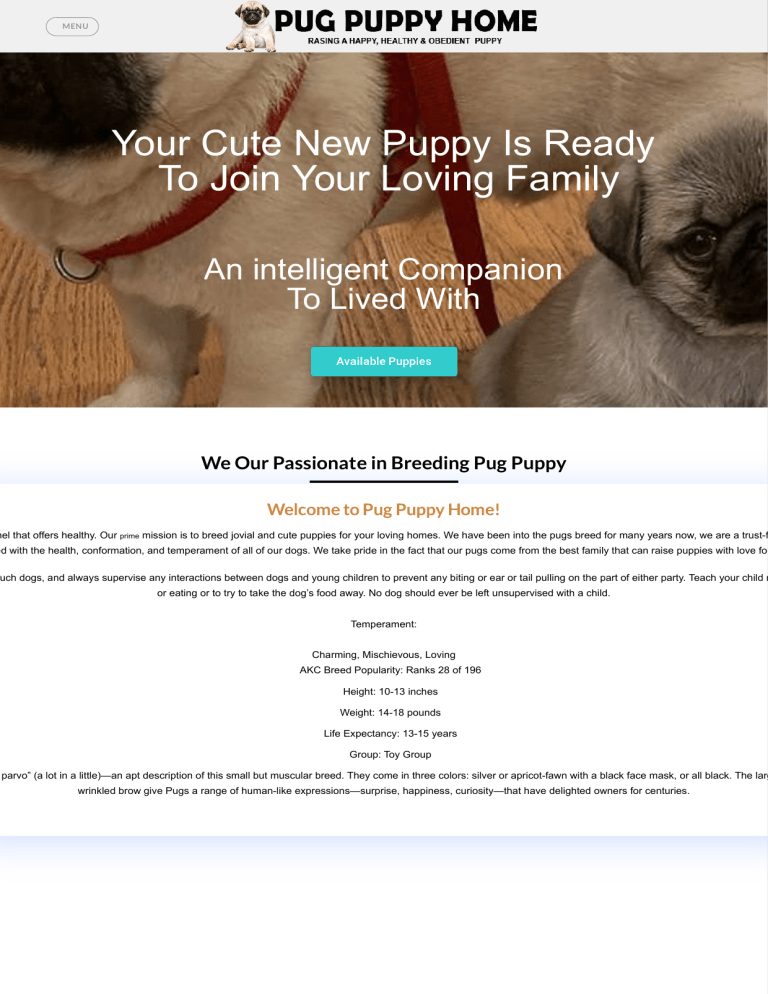This is a detailed caption for the given image:

"This is a screenshot of the website 'Pug Puppy Home.' The byline reads 'Raising a happy, healthy, and obedient puppy.' To the right, there is an image of an adorable pug puppy. Beneath it, there is another image featuring two pug puppies, although part of their faces is cut off. The image is slightly dimmed to enhance the visibility of the white text overlay, which reads, 'Your cute new puppy is ready to join your loving family. An intelligent companion to live with.' Below this text, there is a blue rectangle that says 'Available Puppies.' Further down, there is text that begins with a section emphasizing the website's commitment: 'We are passionate in breeding pug puppies.' Below this, in yellow font, it welcomes visitors with 'Welcome to Pug Puppy Home.' The screenshot appears to be incomplete as some text and parts of the webpage are cut off, but it generally outlines the website's mission, what they offer, and the types of puppies they have available."